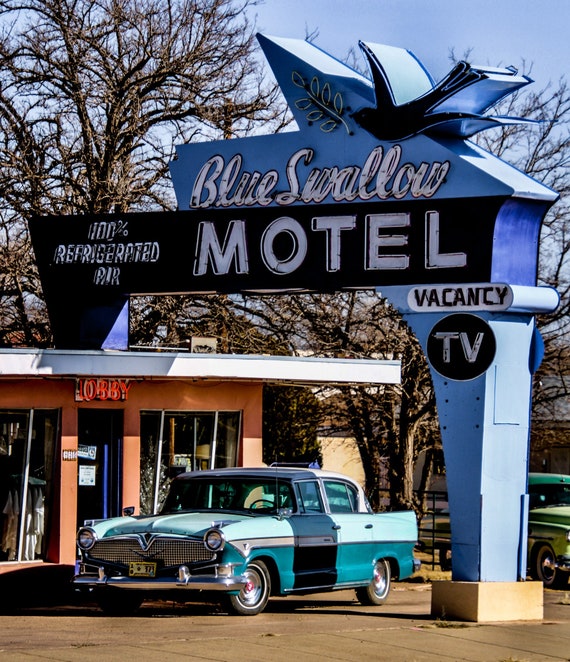This image is a detailed, vintage scene of the front of a 1950s-style motel, captured at an angle. Dominating the foreground is a classic car, elegantly painted in teal and light blue with a white roof, parked under a distinct arching blue sign. This sign, which serves as a focal point of the image, is attached to the one-story lobby building of the motel. The arch extends from the concrete and rises up to the roof, giving it an iconic look. The sign prominently displays the name "Blue Swallow Motel" in cursive, with the word "Motel" in all caps underneath. Additionally, the sign features a small emblem of a bird carrying a leaf, which is either dark blue or black, positioned at the top.

To the left of "Motel," the sign reads, "100% Refrigerated Air," while to the right, smaller signs indicate "Vacancy" and "TV." The lobby building itself is a simple, flat-roofed, rectangular structure painted in an orange hue, with a white overhang. Above the door, in striking red neon, the word "Lobby" is displayed in capital letters. In the background, leafless trees suggest a winter or post-winter setting, with a crisp blue sky overhead, enhancing the nostalgic mood of the scene.